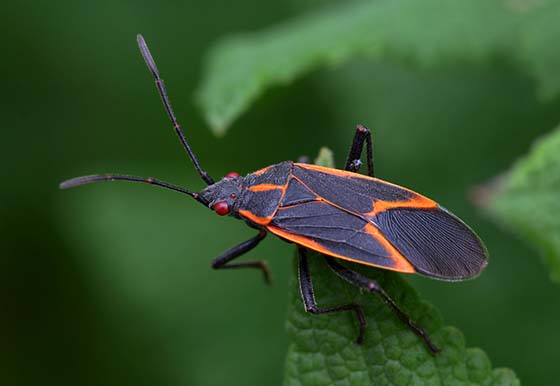This is a close-up photograph of a black insect perched on a vibrant green leaf surrounded by blurred plant life. The bug, which has a distinctive long, oval-shaped body like a firefly or cockroach, is facing west. It features striking red eyes with black pupils on each side of its triangular head, and there is a red dot between the eyes. The black wings are outlined with a vivid orange color that gives them a segmented appearance, almost like delicate cracks. The insect also has six black legs, though only four are clearly visible, and two long black antennae with specks of orange extend from its head. The image composition highlights the bug and the leaf it is perched on, while the rest of the greenery fades into a blurred backdrop, emphasizing the natural setting without specifying the exact location. The bug appears poised, as if ready to jump or fly off the leaf at any moment.